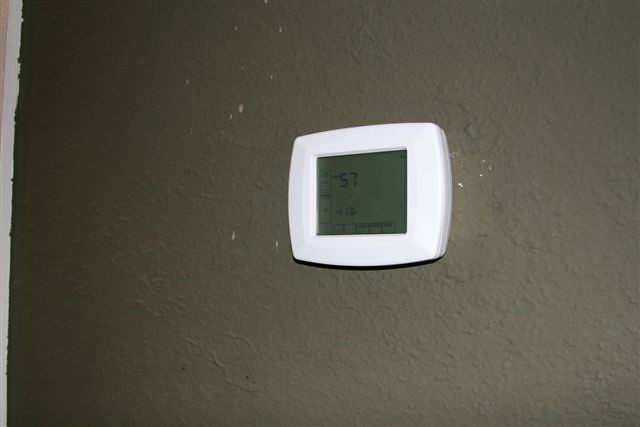The image depicts a grey wood chip wall with a textured surface, featuring visible imperfections such as small grey splatters and approximately ten unpainted chips, mostly around the center of the image. Mounted centrally on the wall is a broadly shaped, rectangular plastic device, presumed to be a thermometer. The thermometer, about half a centimeter thick and with rounded edges, houses a square LCD display showcasing the digits "57". The display also includes unspecified vertical and horizontal graph-like markings. On the left side of the image, a jagged white border, possibly representing an adjoining wall, transitions unevenly into the grey wall, with detectable grey paint overlapping onto the white. In the top left corner, this white border connects to a light brown section, adding a third color to the multi-hued wall.